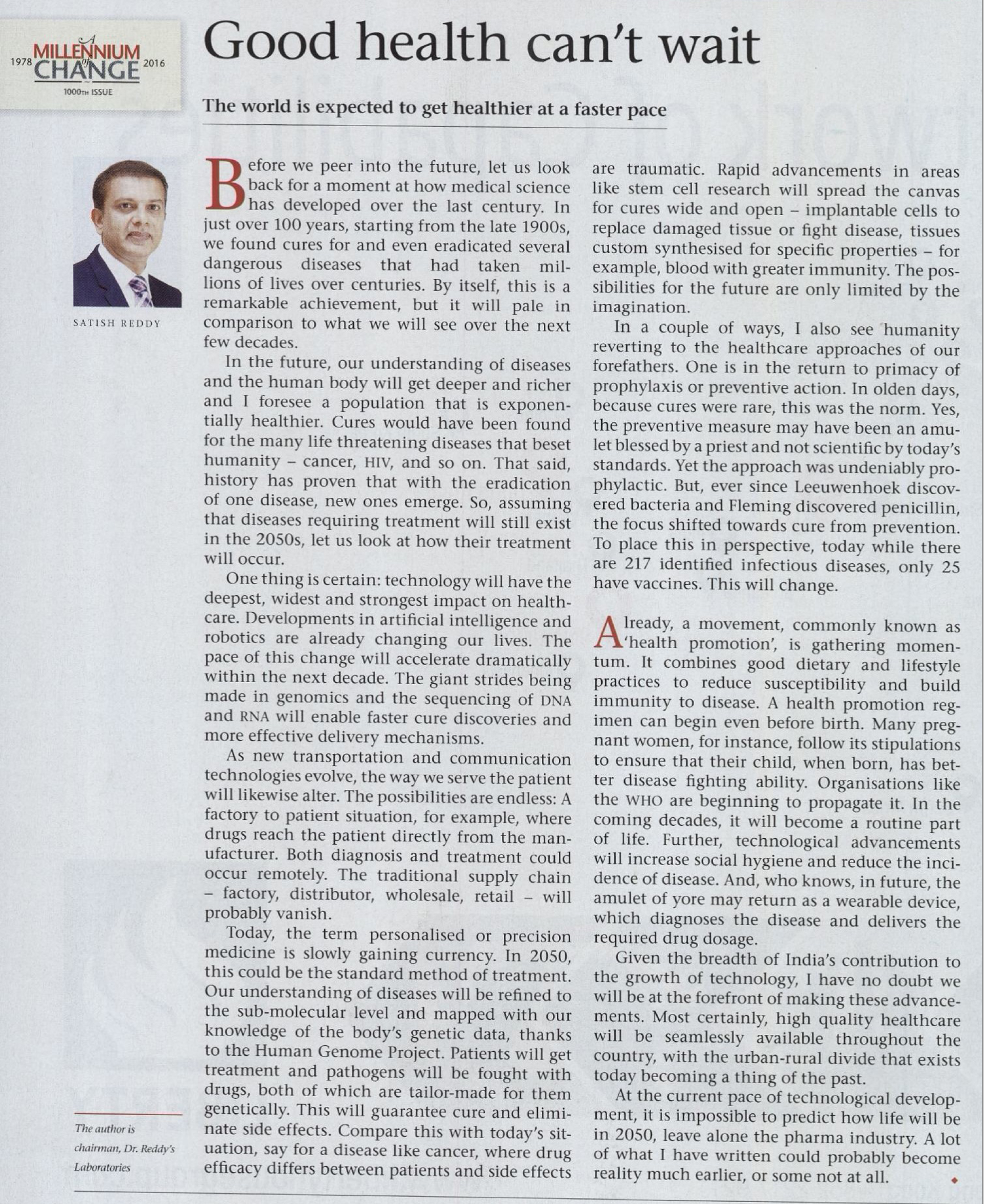The image showcases a print media article, seemingly from the year 2016, with a predominantly grey background. At the top of the page, bold text reads "Good Health Can't Wait." Below this headline, a subheading in bold, underlined text states, "The world is expected to get healthier at a faster pace."

The body of the article is presented in two columns filled with paragraphs of text. The initial letter "B" in the word "Before" is highlighted in a large, bold red font, while the rest of the article is composed in small black lowercase font. Approximately three-quarters through the article, on the second column towards the bottom, another capital letter "A" in red font appears in the word "Already".

On the left side, an empty column features a colored box at the top with the words "Millennium of Change." Additionally, a small font indicates that this is the 1000th issue, though the text is difficult to discern. The word "Millennium" is in the same red font as the prominent letters within the article, while "Change" is displayed in grey, uppercase letters. Adjacent to this text, "1978" is placed on the left and "2016" on the right.

Beneath this summary, there is an image of a man in a suit with dark hair identified as Satish Reddy. Finally, near the bottom of the page, a red line stretches across, with a small italicized caption beneath that reads, "The author is Chairman of Dr. Reddy's Laboratories."